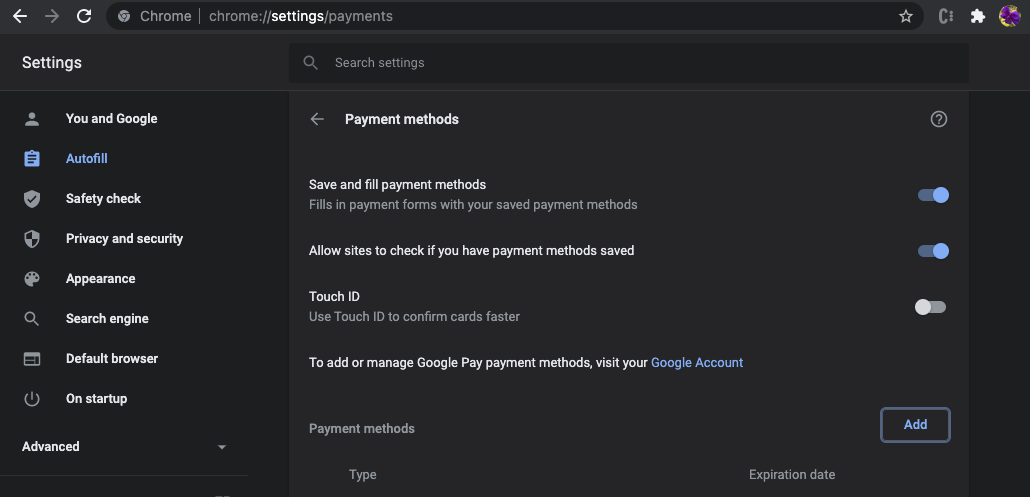Detailed caption: 

The image displays a Google Chrome settings page that features a dark theme with shades of black and dark gray. On the left side, there is a white arrow pointing to the left and a gray arrow pointing to the right. Adjacent to these arrows, a 3-quarter circular white arrow icon is visible, accompanied by a black banner displaying the word "Chrome" in gray text. The URL "chrome://settings/payments" is shown prominently.

Towards the right of the banner, there is a gray star outline and a small profile picture icon. Below this, the "Settings" title is shown in white text. The main menu features several options listed in white text: "You and Google," "Autofill," "Safety Check," "Privacy and Security," "Appearance," "Search Engine," "Default Browser," and "On Startup," each accompanied by a white icon. The "Autofill" option stands out in blue with a blue notebook icon, which has dark brown horizontal lines.

At the very bottom left of the menu, a dark black banner with the word "Advanced" and a downward-pointing arrow is visible. At the top center of the page, a search bar labeled "Search Settings" in gray is displayed, complete with a gray search icon.

Underneath the search bar, the phrase "Payment Methods" appears in white with a left-pointing arrow and a question mark inside a circle on the far right. Below, in white text, it says "Save and Fill Payment Methods," and in gray, it reads "Fills and Payment Forms with your saved payment methods." Accompanying this text, a blue toggle switch is turned on.

The next option, "Allow Sites to Check if You Have Payment Methods Saved," also features a blue on-toggle switch. Following that, "Touch ID" is listed with the description "Use Touch ID to Confirm Cards Faster." This toggle switch, positioned to the left, is off and white. Further down, there is a message reading "To Add or Manage Google Pay Payment Methods, Visit Your Google Account," with "Google Account" in blue text.

At the bottom of the list, the "Payment Methods" section displays columns for "Type" and "Expiration Date." To the far right, an outlined blue square contains the word "Add" in blue text.